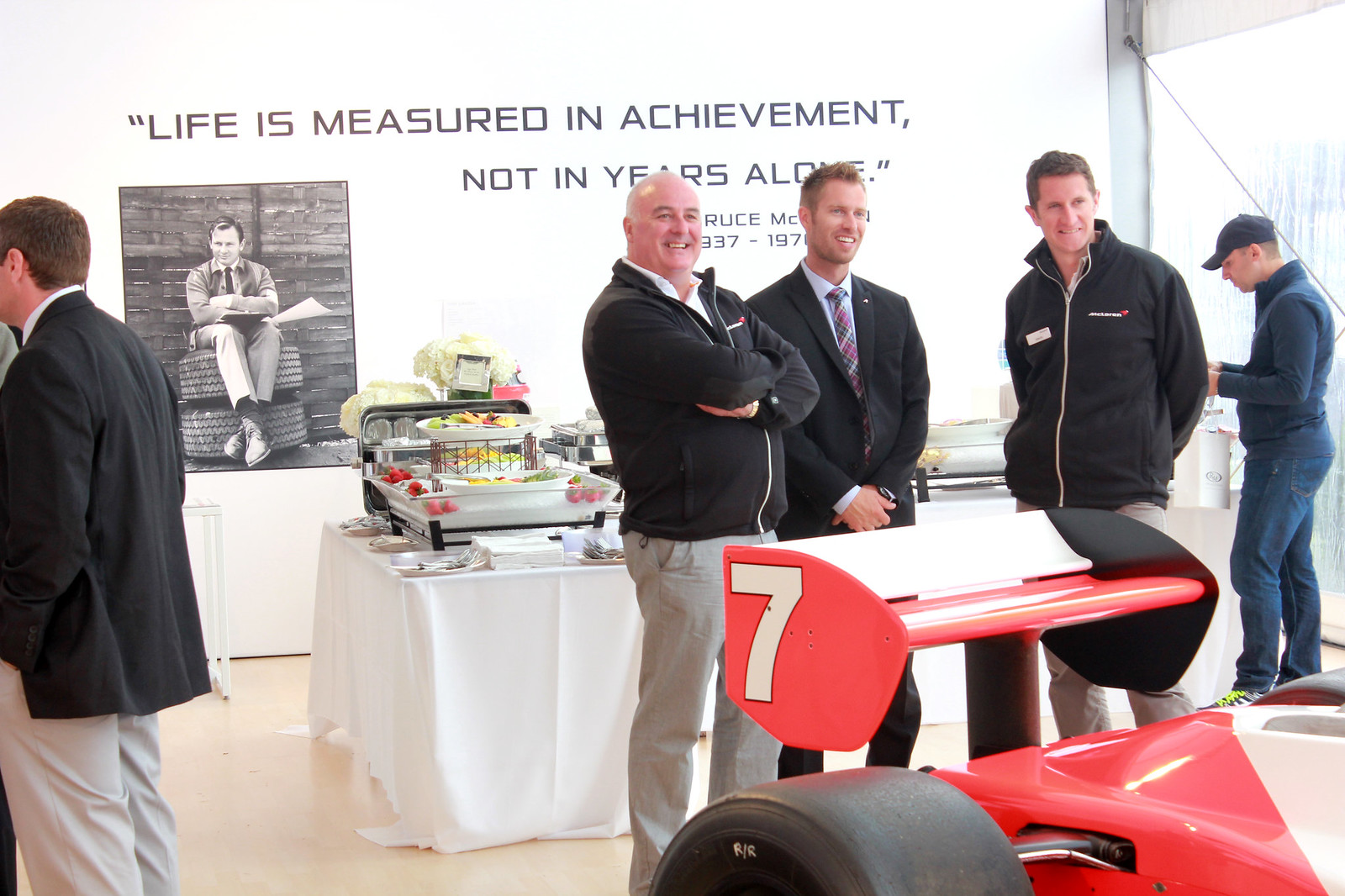In a vibrant showroom, a striking red McLaren race car with a prominent red spoiler emblazoned with the number 7 commands attention. Behind it, three men pose confidently, all smiling and looking in the same direction. The man in the center, appearing to be in his 20s, wears a suit and tie, exuding a professional charm with his short, medium-length hair. To his left stands an older, bald man in a jacket and light pants, distinguished by dark eyebrows and crossed arms. The man on the right sports a dark McLaren track jacket and name tag, with dark hair and light pants, hinting at a possible connection to the distinguished car brand. 

Behind them, the wall bears an inspiring quote: "Life is measured in achievement, not in years alone," attributed to Bruce McLaren, and includes a black-and-white picture of McLaren himself sitting on a stack of tires. The table behind the men displays an array of light refreshments, suggesting a celebratory event or reception. In the background, other attendees meander, adding to the lively atmosphere of the showroom.